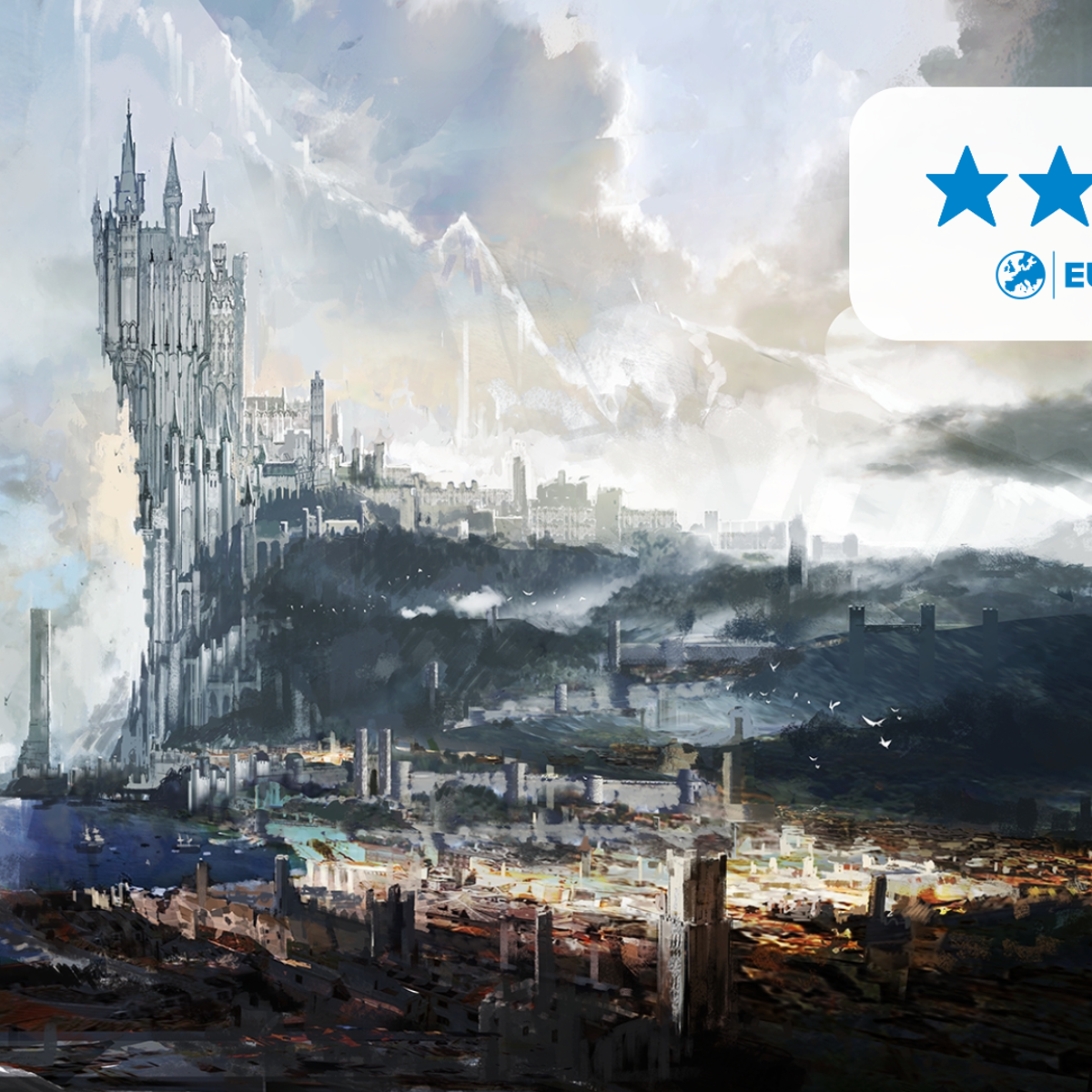The image is an abstract painting depicting a chaotic scene in a city being ravaged by a natural disaster. Massive, tumultuous waves flood the area, covering parts of the cityscape. In the foreground, a towering building—reminiscent of a giant castle or temple—dominates the left side, with white smoke billowing from its damaged structure and three spires reaching into the cloudy sky. The sky itself is a blend of light blue patches, especially in the upper right corner, and various shades of gray, white, and light purple clouds. The city below appears partly submerged in the floodwaters, with smaller buildings scattered throughout and the suggestion of a forest in the background. Artistic elements, such as blue stars in the upper right and the surreal arrangement of waves, clouds, and smoke, add to the abstract and dramatic nature of the scene.